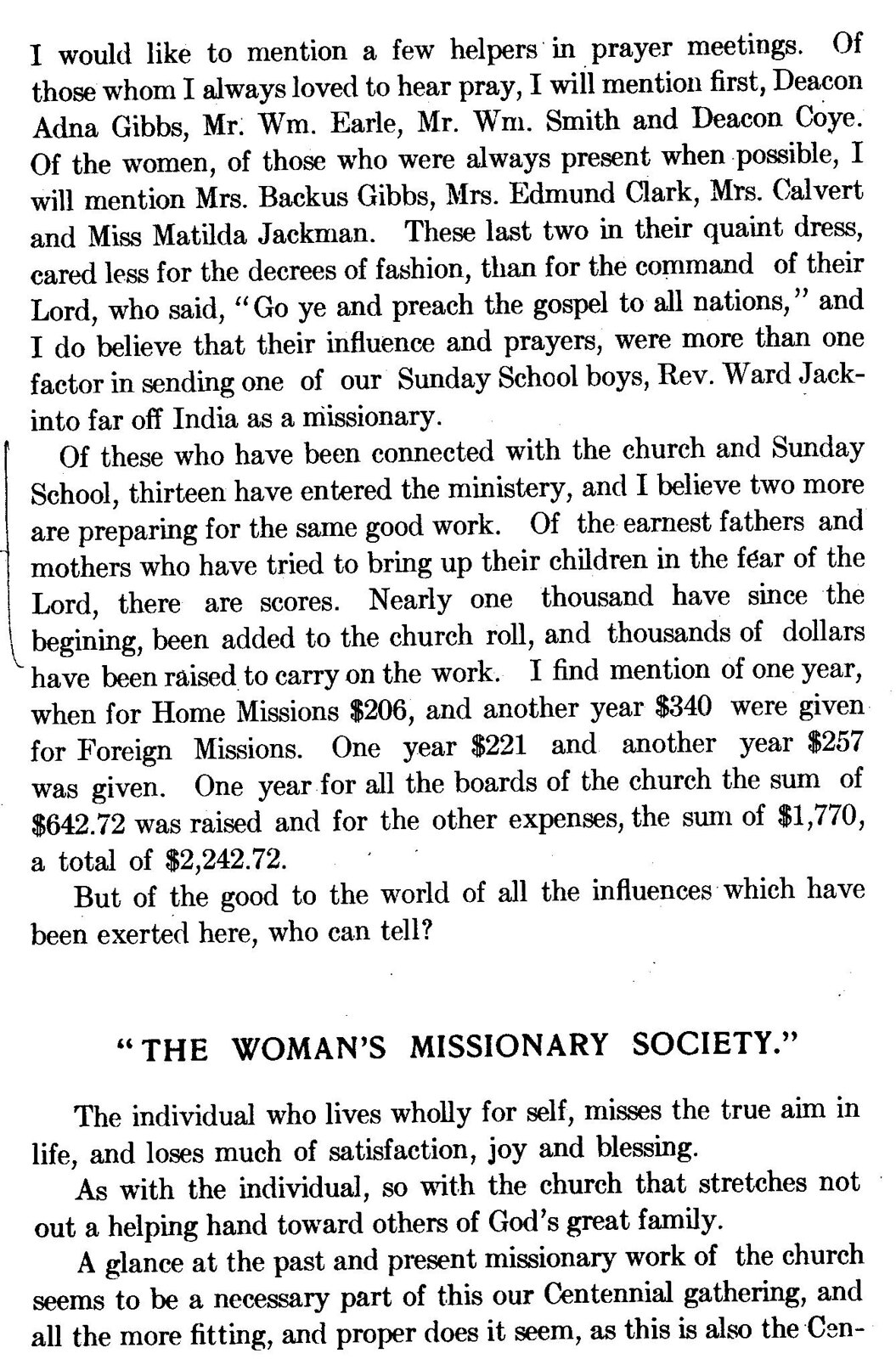This is a black-and-white scan, likely from a newspaper, magazine, or book, which commemorates key contributors to prayer meetings, mentioning both men and women. The text highlights admired male participants including Deacon Adna Gibbs, Mr. W.M. Earl, Mr. W.M. Smith, and Deacon Coy, as well as dedicated female attendees such as Mrs. Bacchus Gibbs, Mrs. Edmund Clark, Mrs. Calvert, and Miss Matilda Jackman. It notes the significant influence of these women, particularly in their contribution to encouraging a Sunday school boy, Reverend Ward Jack, to embark on missionary work in India. Further mentioned is the impact of the church's efforts, stating that 13 members have entered the ministry and two more are preparing. Financial contributions for mission work are detailed, showcasing significant amounts raised for both domestic and foreign missions. The page also mentions the Women's Missionary Society, emphasizing the importance of selflessness in achieving true satisfaction and the integral role of missionary work in the church's centennial celebrations.